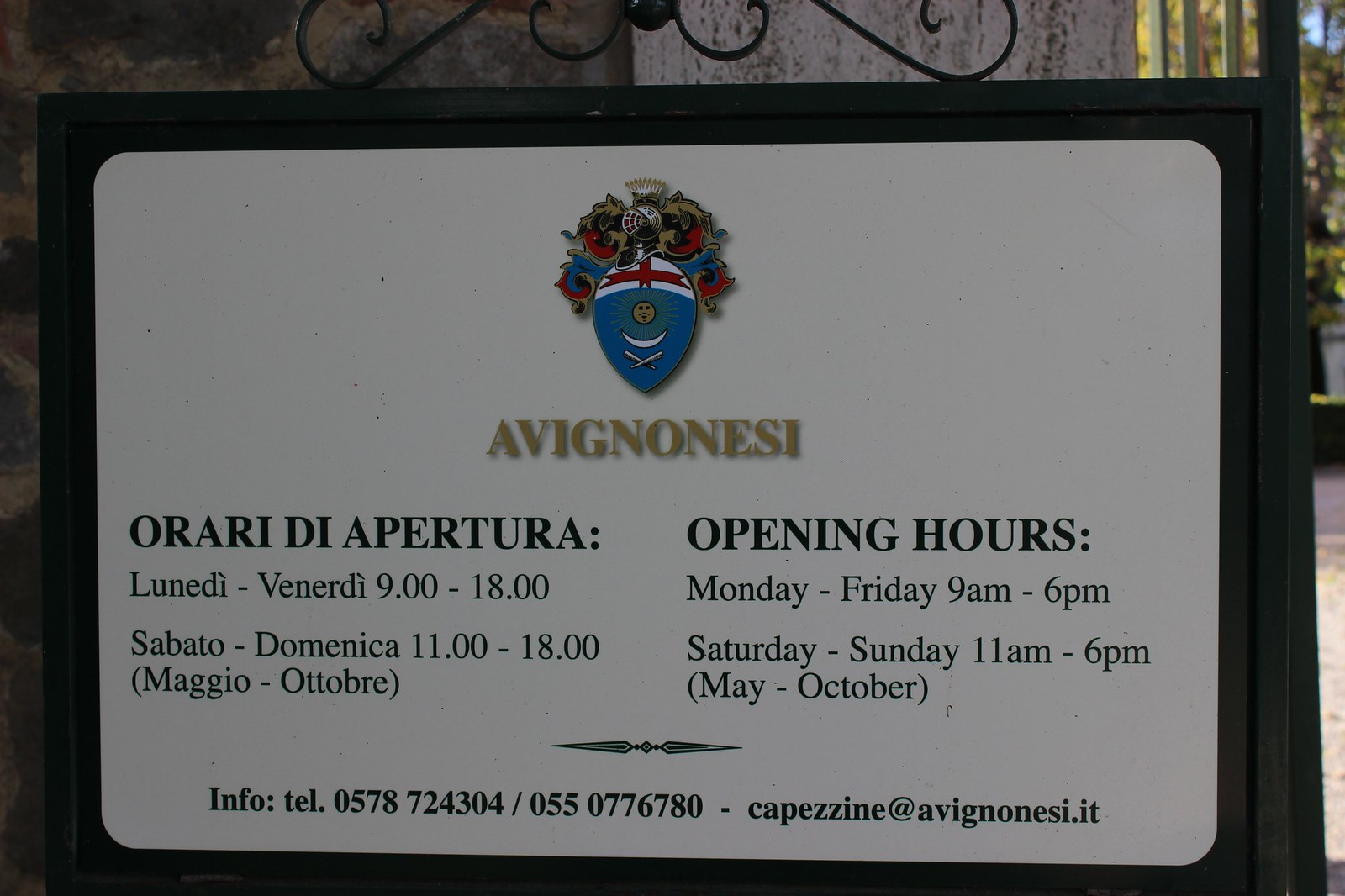The image depicts an outdoor sign attached to a gate, set against a bright and clear background, reflecting natural light. The sign features a prominent crest at the top, incorporating a blue, white, red, and yellow design. The crest includes a sun, a moon, and two crossed sticks beneath what appears to be a knight's helmet.

Beneath the crest, the word "Avignonesi" is clearly displayed. The left side of the sign is likely in Italian, displaying the opening hours as "Orari di Apertura," and the right side translates this information into English. It states the opening hours as follows: Monday through Friday, 9 a.m. to 6 p.m., and Saturday and Sunday, 11 a.m. to 6 p.m., for the period of May to October.

At the bottom, the sign provides contact information, listing a telephone number, 0578-724-304/055-0776-780, and an email address, CAPEZZINE@AVIGNONESI.IT. This comprehensive information indicates that the sign is related to Avignonesi, likely an Italian establishment, given the URL suffix and the language used.